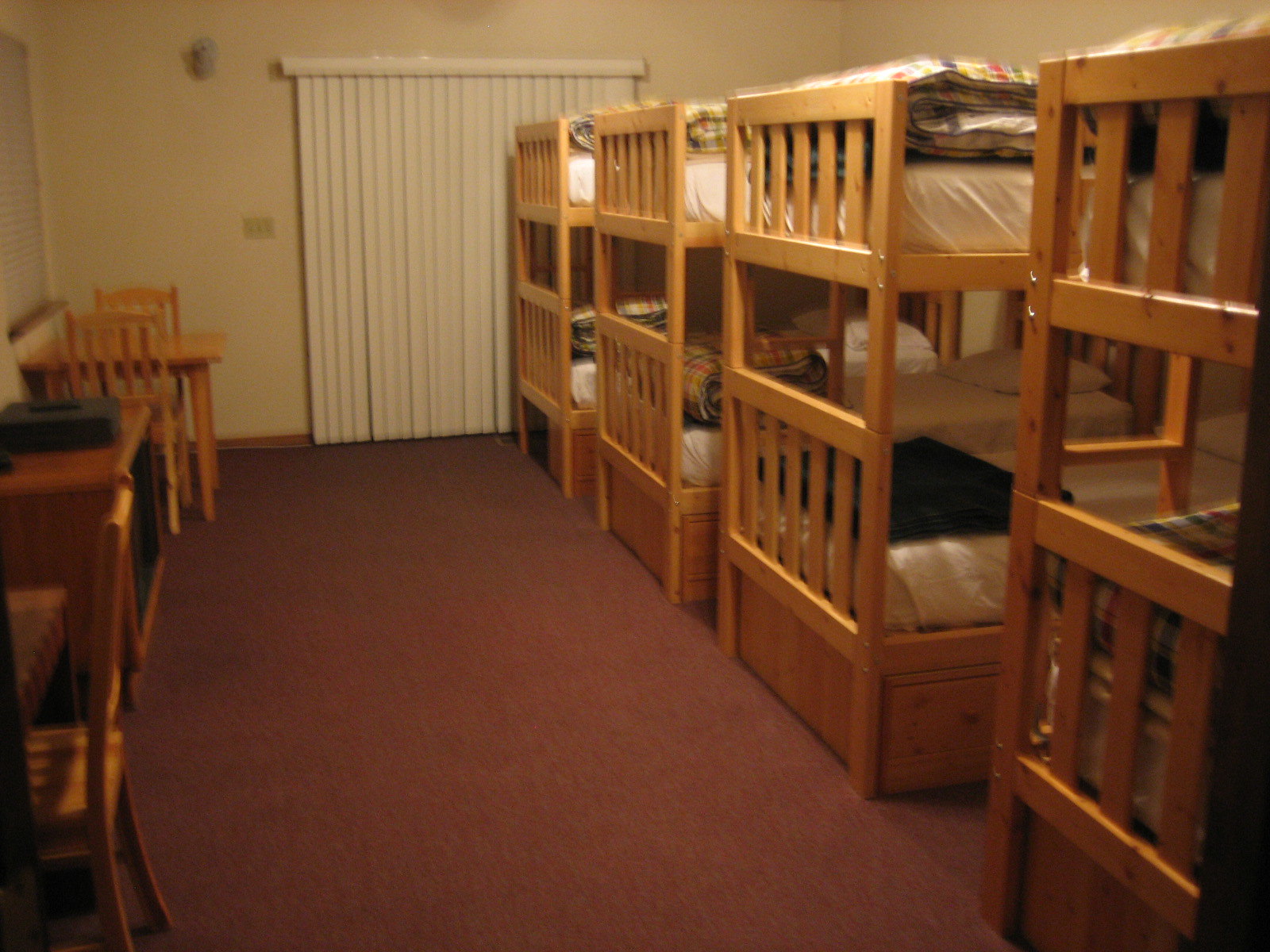The photograph captures a dormitory-style bedroom with a light yellow or beige wall and a maroon carpet. On the back wall, there's a large window or sliding glass door covered by closed white vertical blinds. On the right side of the room, there are four sets of wooden bunk beds, each equipped with white sheets and varying blankets. Most of the blankets are plaid with red, yellow, and blue stripes, while one bed has a black blanket. Each bed also has a folded comforter at the foot. The left side of the room features two small wooden tables accompanied by three wooden chairs, arranged in a way that one table has two chairs and the other has one. There is also a dresser or cabinet between the tables. Light from an unseen source illuminates the bunk beds, enhancing the cozy yet simple atmosphere of the room.